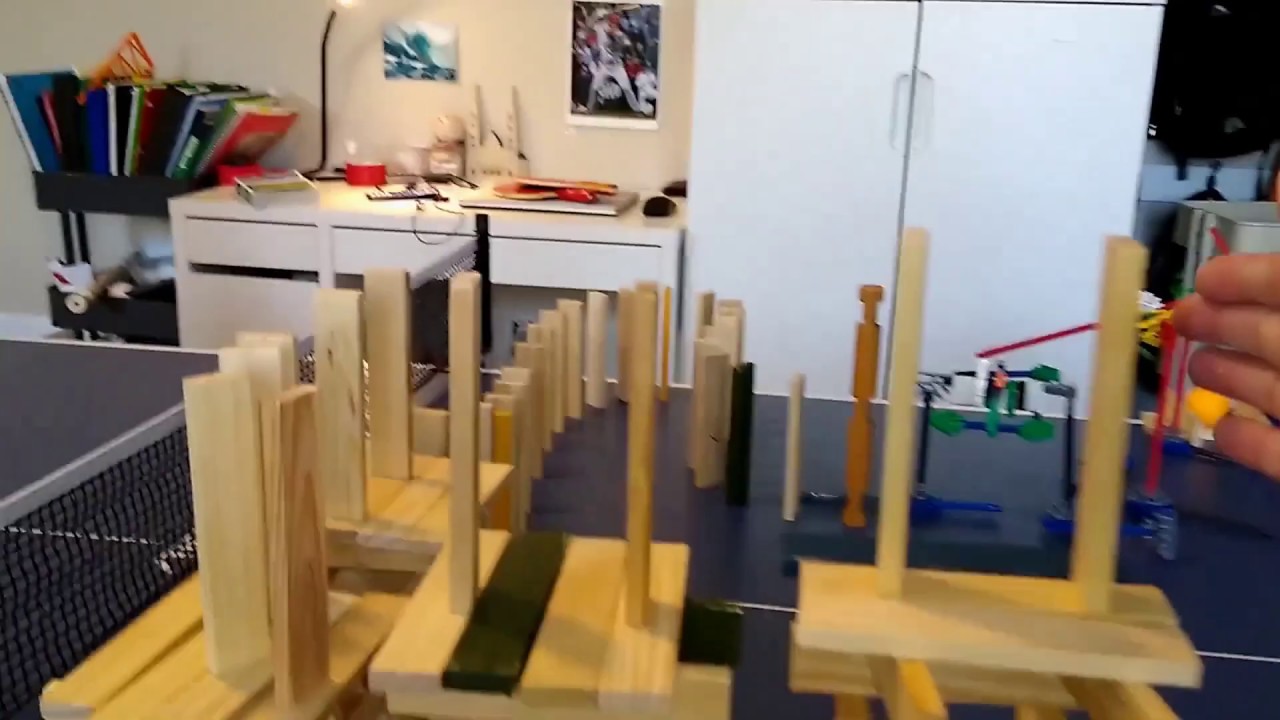The image depicts a cluttered room with a prominent impromptu domino setup in the foreground. On the left side, there's a white desk cluttered with various items, and above it hangs a poster of a baseball player in a grey uniform with a red helmet. Adjacent to the desk is a black cart overflowing with tall books. To the right, there's a tall white cabinet with smooth door fronts. Dominating the foreground is a blue-black table tennis table, with a black net featuring a white stripe running from the bottom left corner to about two-thirds of the way across. The right half of the table is occupied by a complex domino setup made of stacked small wooden rectangular prisms. These prisms form high structures at the bottom right, progressively declining in layers towards the center and further back. Vertically standing wooden prisms follow this descending path. Toward the far right of the image, a blurred set of four fingers is poised to interact with the rightmost domino piece, suggesting imminent action.